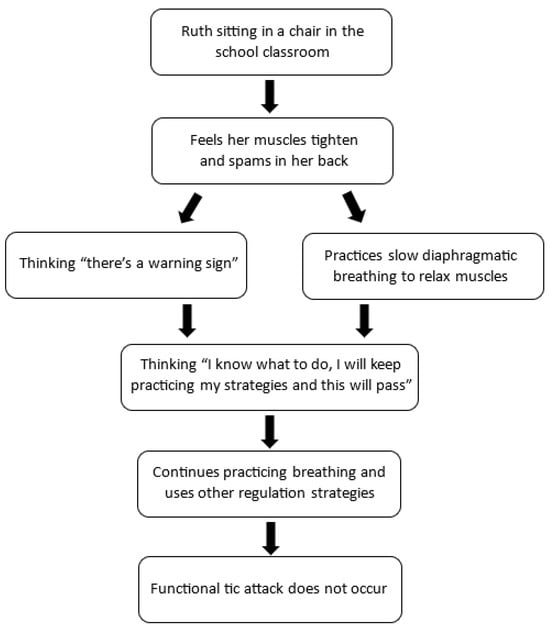This image is a detailed flow chart designed to help manage muscle spasms and potential tic attacks, commonly associated with Tourette's syndrome, particularly in a school setting. It presents a sequence of actions and thoughts in black text on a white background, with rounded-corner rectangles and black arrows connecting each step.

1. The top rectangle reads: "Ruth sitting in a chair in the school classroom."
2. A downward arrow points to another rectangle: "Feels her muscles tighten and spasms in her back."
3. From this rectangle, arrows branch out diagonally:
   - To the left: "Thinking, 'There's a warning sign.'"
   - To the right: "Practices slow diaphragmatic breathing to relax muscles."
4. Both of these rectangles lead to a common rectangle below with the text: "Thinking, 'I know what to do. I will keep practicing my strategies and this will pass.'"
5. Another downward arrow follows to the next rectangle: "Continues practicing breathing and uses other regulation strategies."
6. Finally, a downward arrow from this rectangle leads to the last box: "Functional tic attack does not occur."

Overall, the flow chart serves as an educational tool to guide individuals, particularly those with Tourette's syndrome, through a series of cognitive and physical strategies to prevent or mitigate tic attacks.